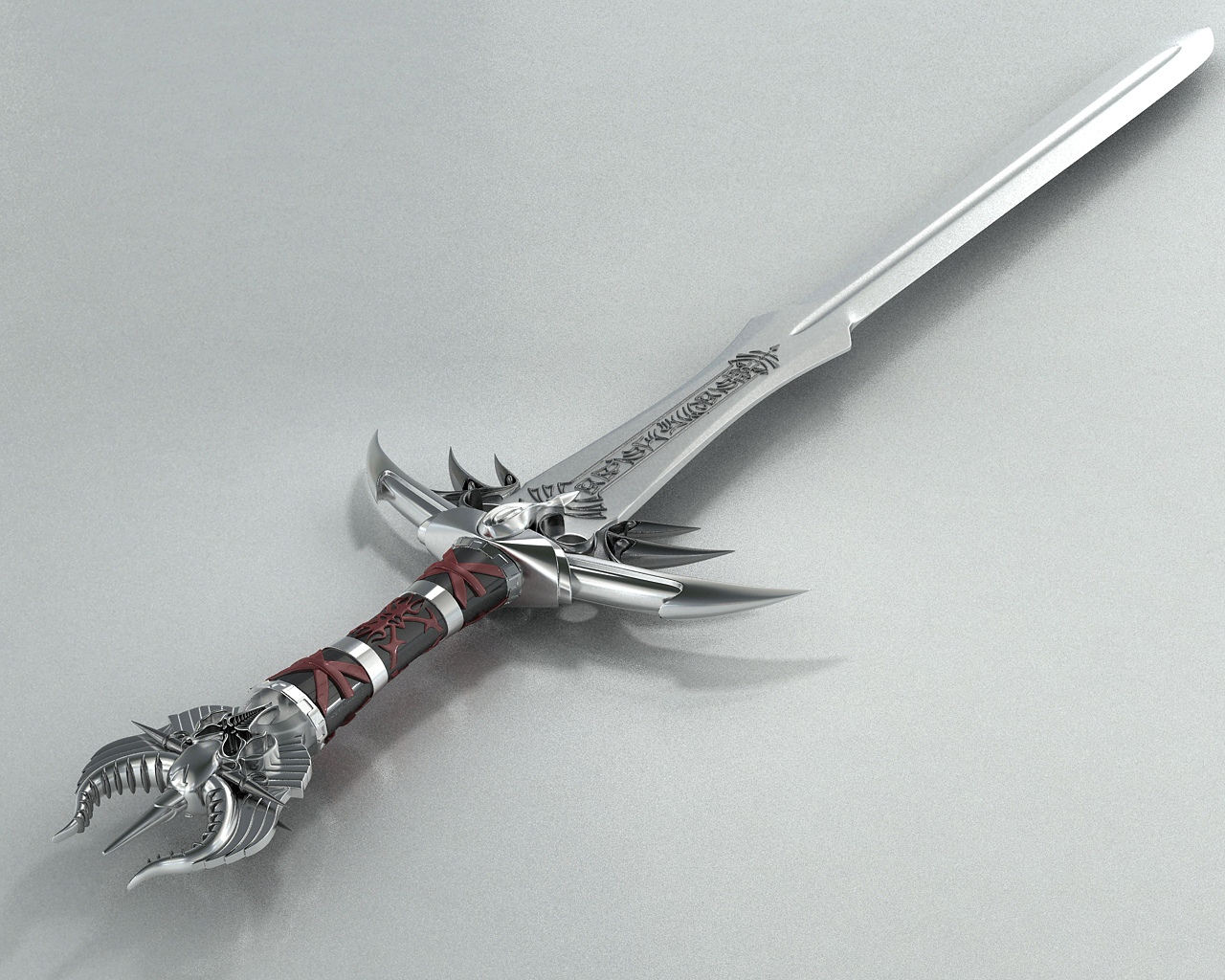This photograph captures an ornate, full-sized sword set against a white background, possibly on a table. The sword features a long, silver blade adorned with intricate black designs that include Chinese symbols. The handle is a striking combination of red, black, and silver, embellished with three distinct red symbols. The bottom of the handle boasts a large, ornate silver design. Unique and striking, the handle is equipped with sharp prongs: three on each side where one's hand would grip and three more protruding from the back. The overall appearance is imposing and sharp, with the blade extending diagonally from the lower left to the upper right of the image.